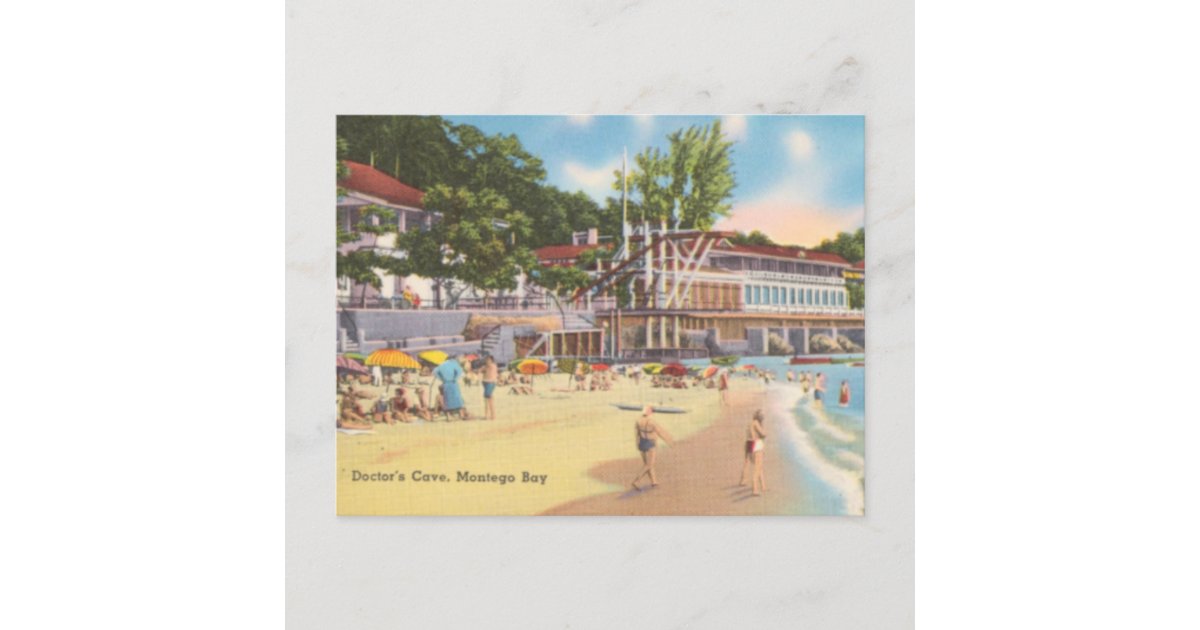This image features a photograph of a postcard, placed on a light gray marble countertop with subtle gray streaks. The postcard, approximately 1.5 inches wide and 1 inch tall, captures a vibrant beach scene at Doctor's Cove, Montego Bay, which is labeled in gray print on the lower left-hand corner. The scene showcases a sandy beach populated with numerous people sitting under umbrellas, some wading in the blue ocean water, and others walking along the shore. In the background, lush green trees frame a resort area, including a prominent hotel-like structure supported by circular stilts and perhaps an outdoor awning for picnicking. Above the picturesque beach, the sky is a bright blue adorned with fluffy white clouds, casting a serene and inviting atmosphere over the entire scene. The postcard itself is bordered by a thicker gray boundary on the top and bottom, enhancing its framed appearance on the countertop.